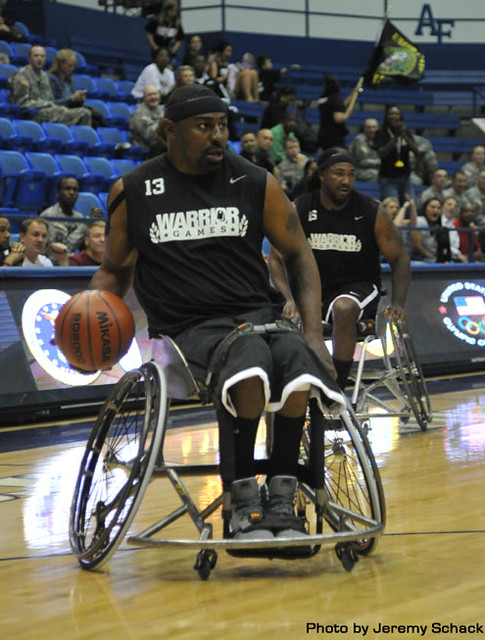In the midst of a thrilling wheelchair basketball game, a dynamic scene unfolds on a bustling court. The central focus is on an athlete donning a black sleeveless jersey emblazoned with "Warrior Games" and sporting the number 13 on his right shoulder. Complementing his attire, the player wears black shorts, a black cap, a black headband, and gray tennis shoes with black socks. Maneuvering his specially designed sports wheelchair with his left hand, he skillfully balances a basketball in his right.

This player, characterized by his short black hair and tattoos, epitomizes strength and determination. Positioned behind and to his right, another player, identifiable by his similar uniform and the number 35 on his chest, also engages intensely in the game. Both athletes, marked by their black and white uniforms complete with Nike logos, navigate the court in purpose-built wheelchairs designed for competitive play.

The background buzzes with vibrant energy, as spectators fill the blue-seated bleachers. Some fans stand, others sit engrossed in the game, and one, slightly blurry, waves a flag. The court itself is clearly visible at the bottom of the image, bordered by barriers that separate the players from the crowd, adorned with various logos. The environment echoes the competitive spirit and camaraderie of a true sports spectacle.